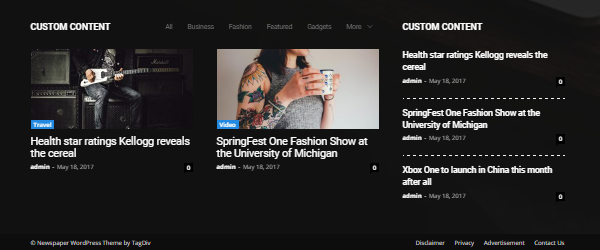The image presented appears to be a screenshot of a website, characterized by a black background and featuring a 2.5:1 width-to-height ratio. At the top center, the website showcases a horizontal menu with small gray text options, including "AI," "Business," "Fashion," "Featured," "Gadgets," and potentially others. On the upper left corner, larger white text reads "Custom Content."

The content is divided into sections. The first section features an image of a man dressed in black, seated on a chair, and playing a black and white guitar. Below this image, bold white text states, "Health Star Ratings, Kellogg Reveals the Cereal."

Adjacent to the first image, towards the right, is another section showcasing a close-up image of a woman's chin and chest area, angled around a 5 o'clock direction. The woman has her right arm, which is adorned with multiple tattoos including designs of a sun and a star, bent upwards so her hands are cradling a cup, possibly a coffee cup, in front of her chest. Below her image, bold white text reads, "Spring Fest, One Fashion Show at the University of Michigan."